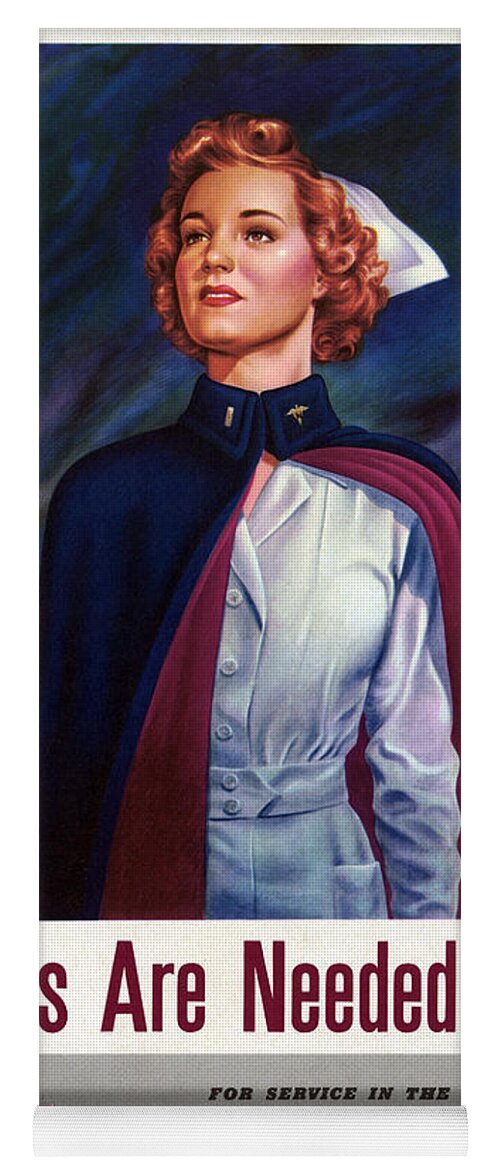This is an illustrated image that likely hails from an old-timey magazine or newspaper advertisement, possibly a military recruitment ad for nurses. The main subject is a fair-skinned young woman in her early 30s, who has short, reddish-golden, curly hair, and is adorned with meticulous makeup featuring rosy cheeks and red lipstick. She is dressed in an old-time nurse’s uniform—a white button-down shirt or dress, which is obscured from the waist down by the image's crop. Draped over her shoulders is a navy blue cape with a dark red lining, securely fastened at the collar with a clasp, revealing medallions on her uniform collar. The nurse's cap atop her head complements her uniform. She stands tall and prominently against a blue background that accentuates her features. Below her, partially visible text reads, “R needed for service in the -,” hinting at a call for nurses, potentially for military service.